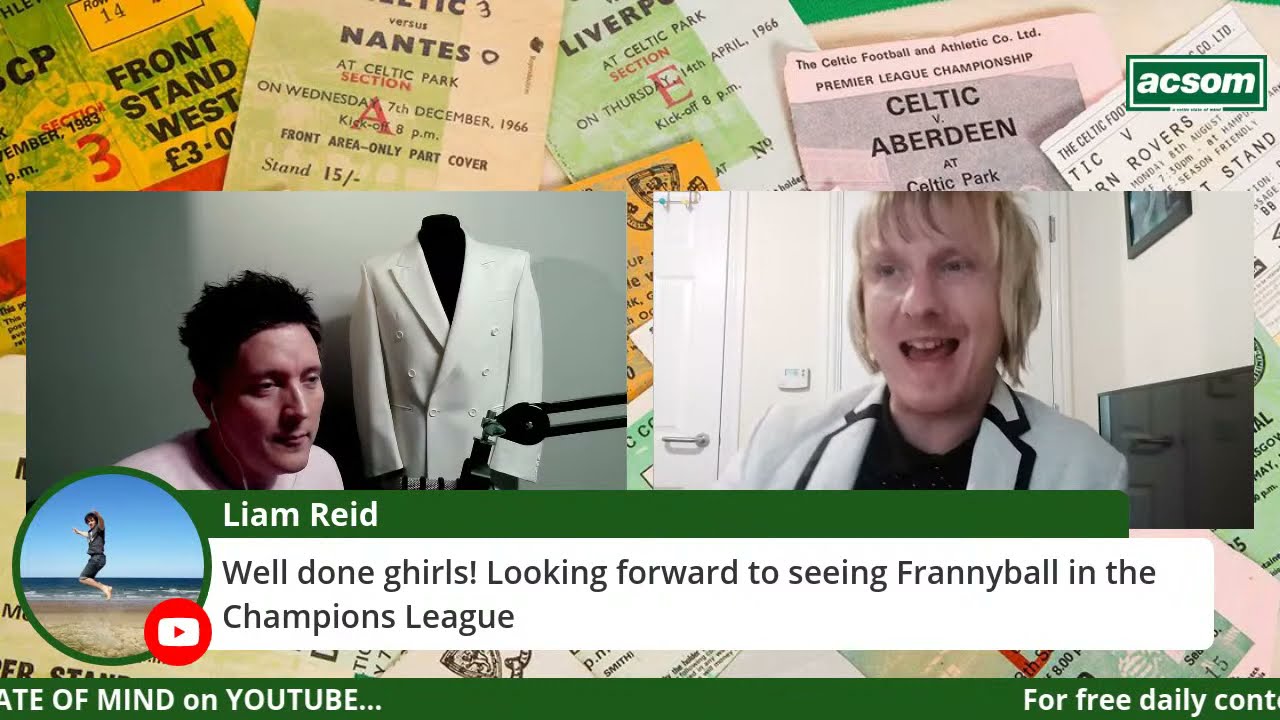This screenshot from a podcast video on YouTube features two gentlemen in separate settings, each participating in a remote discussion. On the left, the dark-haired man is seated in a room with a mannequin draped in a white coat beside him, and a plain white wall in the background. On the right, a blond man, wearing a white coat over a black shirt, is speaking with his mouth open, set against a backdrop of a white wall and some cabinets. Between their images, a horizontal strip displays a comment from a user named Liam Reid, which reads: "Well done girls looking forward to seeing Franny Ball in the Champions League," accompanied by a circular profile picture of Liam Reid. The screenshot also contains scattered images resembling tickets or pamphlets. In the top-right corner, a rectangular logo with the text "Exxon" is visible. At the bottom, a green strip reads “Eight of Mind on YouTube” on the left and “For Free Daily Content” on the right.